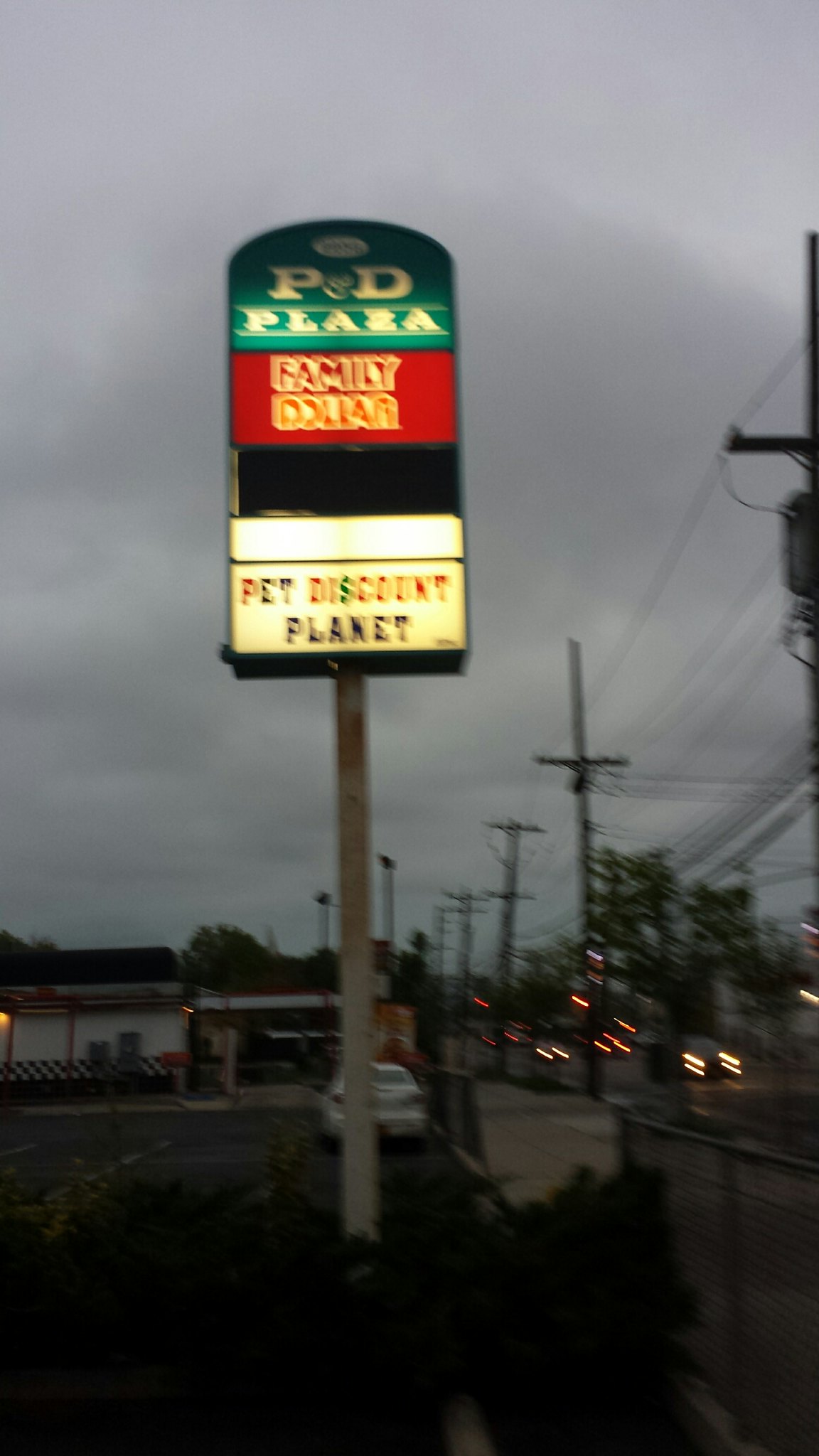In this outdoor photograph taken at dusk, the sky is heavily clouded, suggesting recent or incoming inclement weather. The image prominently features a tall, white post with a shopping center sign. At the top of the sign, illuminated faintly, it reads "P&D Plaza," followed by an orange sign for Family Dollar, and a bottom sign for Pet Discount Planet. The photo appears slightly blurry but reveals additional details: to the left of the sign, a drive-thru restaurant, possibly a Checkers or Riley's, characterized by a white building with checkered patterns, is partially visible. Several cars with headlights on can be seen driving down the adjacent street, and there is a white car parked behind the sign. The overall scene is dimly lit, emphasizing the transitional time between day and night.